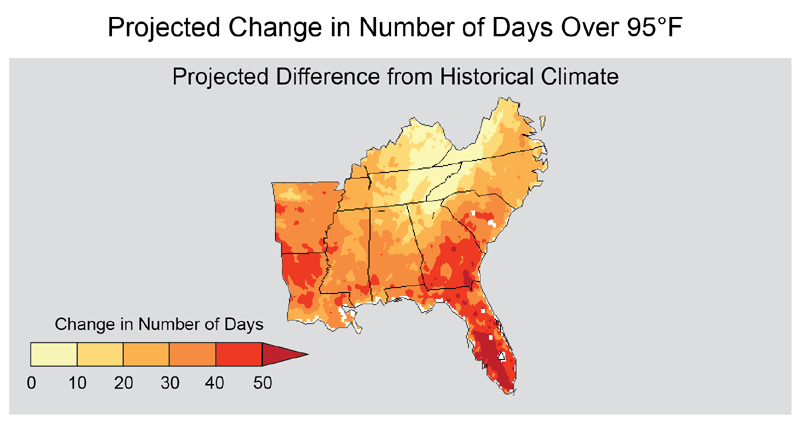This is a detailed graphical heat map of the southeastern United States, showcasing the projected change in the number of days with temperatures exceeding 95 degrees Fahrenheit. The title positioned at the top-center reads "Projected Change in Number of Days Over 95 Degrees Fahrenheit" against a white background. Below this, within a boxed gray rectangular area, it states "Projected Difference from Historical Climate." At the bottom left, a color-coded legend spans from yellow to dark burgundy red, indicating the "Change in Number of Days" ranging from 0 to 50. Specifically, light yellow signifies 0 to 10 days, progressing through shades of orange, and culminating in dark burgundy red for 40 to 50 days. The map itself, though not labeled with state names, clearly identifies the southernmost states, notably Georgia and Florida, exhibiting a significant increase in the number of days over 95 degrees. Conversely, the more northern states like Virginia, Kentucky, and parts of Tennessee show minimal to no change, remaining at 0 days. This visual presentation effectively communicates the intensifying heat projected for the southern regions compared to the historical climate data.